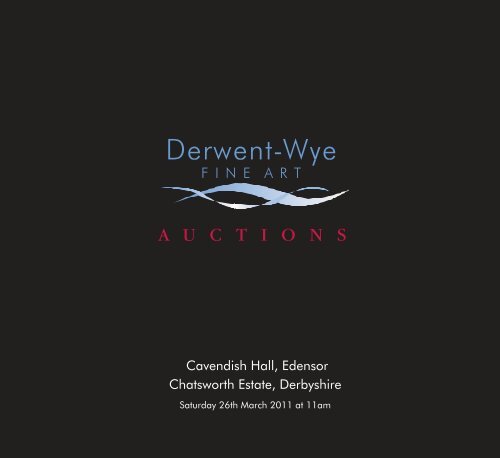The square-shaped advertisement features a solid black background with minimal yet striking text, focusing on an upcoming event. Centered slightly towards the top, in blue font, the text reads "Derwent - WYE Fine Art." Below this, two interwoven ribbons, resembling waves, add a touch of decorative flair. Following the ribbons, the bold red text announces "Auctions." Further down, in smaller white font, three separate lines detail the event's specifics: "Cavendish Hall, Edensor, Chatsworth Estate, Derbyshire." At the very bottom, in even smaller white text, the date and time are given: "Saturday 26th March 2011 at 11 a.m." The advertisement is stark and elegant, with no other illustrations or pictures, relying solely on the contrasting texts and designs against the black background to convey its message.